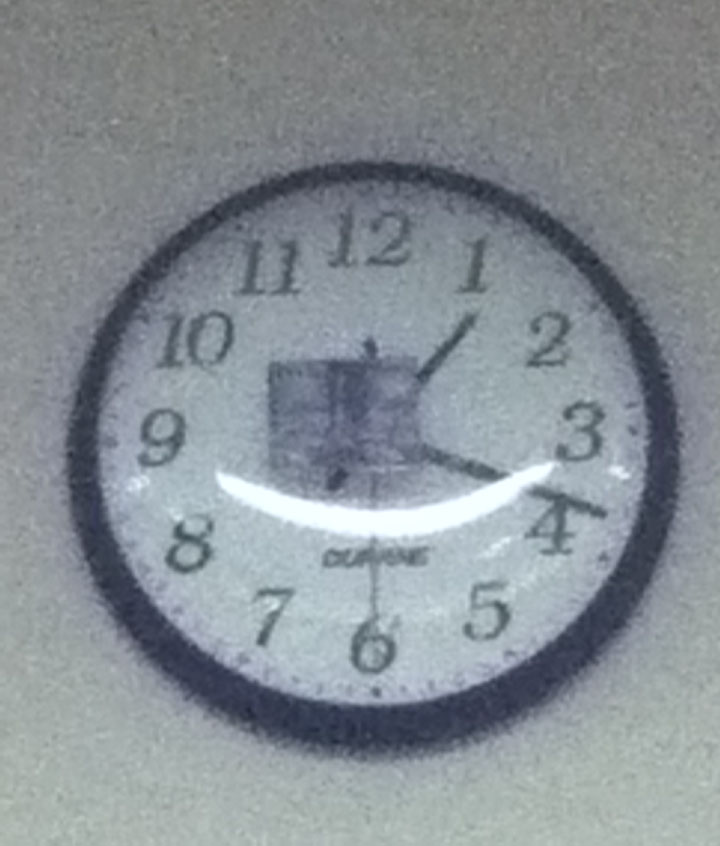This is a grainy, black-and-white photograph capturing an analog clock mounted on a wall. The clock features a white face, with black numerals from 1 to 12 encircling the dial. The hour and minute hands are black, while the second hand appears darker but could potentially be red, given the monochromatic nature of the image. Although the manufacturer’s name, typically positioned beneath the center of the clock hands, is indistinguishable due to the image's poor resolution, there is some kind of picture or emblem in the middle of the clock face that also remains unclear. The black border of the clock contrasts with what might be a white wall in the background, though the graininess of the photograph makes this uncertain. The time displayed is approximately 1:18 and 30 seconds.